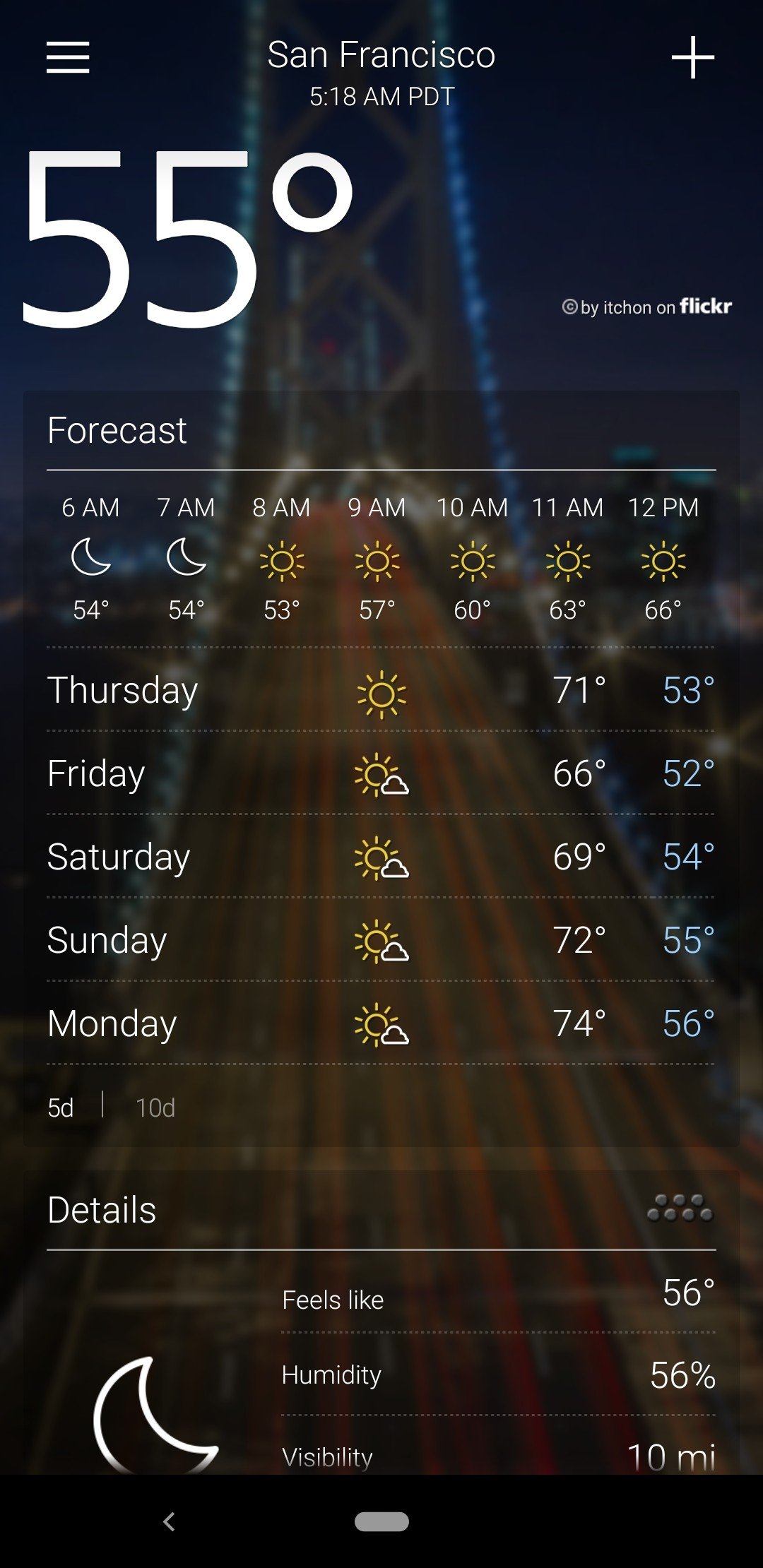The image displays a detailed weather forecast for San Francisco on an Android smartphone. The time is shown as 5:18 a.m. PDT (Pacific Daylight Time) with a current temperature of 55°F. The hourly forecast indicates clear skies, with temperatures gradually rising from 54°F at 6 a.m. to 66°F by 12 p.m.

The extended forecast for the next few days is also included:
- **Thursday**: Sunny with a high of 71°F and a low of 53°F.
- **Friday**: Partly cloudy with a high of 66°F and a low of 52°F.
- **Saturday**: Mostly sunny with a high of 69°F and a low of 54°F.
- **Sunday**: Partly cloudy with a high of 72°F and a low of 55°F.
- **Monday**: Mostly sunny with a high of 74°F and a low of 56°F.

Additional weather information is available at the bottom of the display.